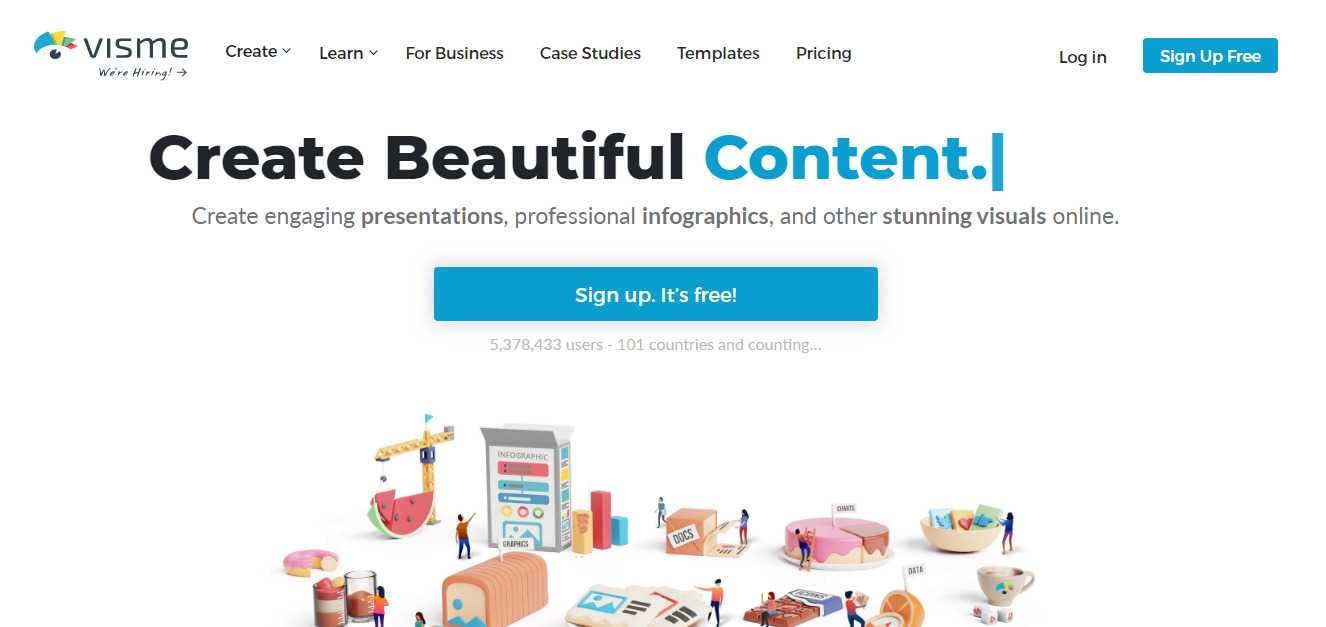The top of the webpage prominently features the word "VISME" in relatively large letters with an icon to its left. Following "VISME" to the right are categories listed in smaller font: "Create," "Learn," "For Business," "Case Studies," "Templates," and "Pricing." Further to the right are options to "Log In" and "Sign Up Free." Below, in very large, bold text are the words "Create beautiful content." The words "Create" and "Beautiful" are in black, while "Content" is in blue, followed by a period. A short line extends slightly longer than the word "Sign Up," emphasizing that the sign-up is free. Beneath this text is a collection of seemingly random images including a watermelon, a crane, a cake, and a teddy bear.